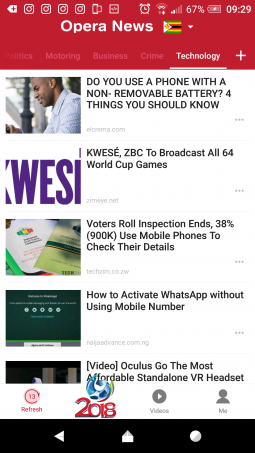At the top of the page is a large red banner with the text "Opera News" prominently displayed. Adjacent to the text is a flag featuring a sideways white triangle, with stripes in green, yellow, red, black, red, and green. Across the top of the page are several white icons indicating 67% battery, the time 09:29, and other status indicators.

Below the banner are several headings in light print, which are difficult to read. The word "Technology" is displayed in white, underlined, with a plus sign next to it. The left side of the page features multiple images:

1. The first image is of a man in a blue shirt, with the caption: "Do you use a phone with a non-removable battery? Four things you should know", followed by a dot-com address.
  
2. The second image showcases large purple text reading "Queezy" and states, "Queezy ZBC to broadcast all 64 World Cup games". The accompanying image shows green and white squares.

3. Another caption reads: "Voters roll inspection ends 38%. 900,000 use mobile phones to check their details".

4. "How to activate WhatsApp without using a mobile number" is another highlighted section.

5. Part of a video about "Oculus Go, the most affordable standalone VR headset" is visible as well.

There is a white box with a red refresh button and a semi-circular blue film icon displaying "2018" in red. Next to it is a gray button labeled "Videos" and an icon resembling "MU" with a little person symbol.

Towards the bottom, a black box contains icons including a white return button, a house symbol, and a circle.